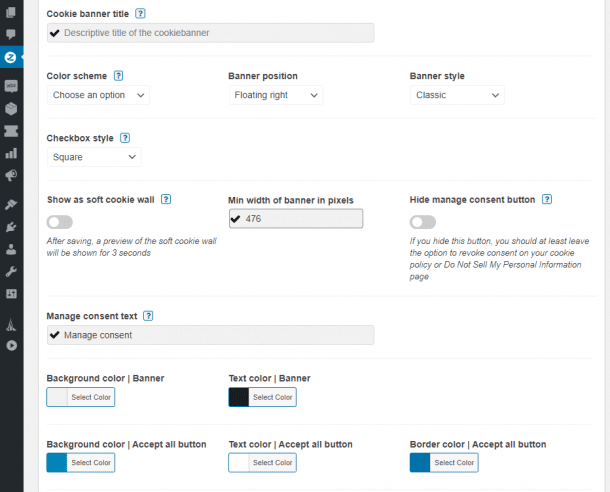This image depicts a configuration interface for setting up a cookie consent banner on a website. The section titled "Cookie Banner Settings" is prominently displayed at the top, enclosed in a blue box with a question mark icon. Below this, it reads "Descriptive Title" for the cookie banner.

Key configuration options and their current settings are as follows:
- **Cookie Sheet Scheme**: Users can choose an option from a dropdown menu.
- **Banner Position**: Selected as "Floating Right" from a dropdown menu.
- **Banner Style**: Set to "Classic," also from a dropdown menu. Other styles can presumably be selected.
- **Checkbox Style**: Displayed as "Square" from the available options.
- **Show a Soft Cookie Wall**: This option is not enabled.
- **Minimum Width (in pixels)**: Set to 476 pixels.
- **Hide Manage Consent Button**: A recommendation is shown advising to leave an option for revoking consent through the cookie policy page if this option is hidden. This checkbox is not checked.
- **Do Not Sell My Personal Information**: This option is also not checked.
- **Manage Consent Text**: The option is checked, enabling this section.
- **Background Color / Banner**: Currently set to a grey shade.
- **Text Color / Banner**: Set to black.
- **Background Color (Accept All Button)**: Configured to a specific shade of blue.
- **Text Color (Accept All Button)**: Set to white.
- **Border Color (Accept All Button)**: A slightly darker blue.

On the left side of the interface, there is a vertical toolbar with several icons, each corresponding to different sections or features of the setup. One of these icons, resembling the letter "Z", is highlighted in blue, indicating the current selection or focus.

Overall, the image provides a detailed view of the various customizable settings available for creating and managing a cookie consent banner, including styling and positioning options.